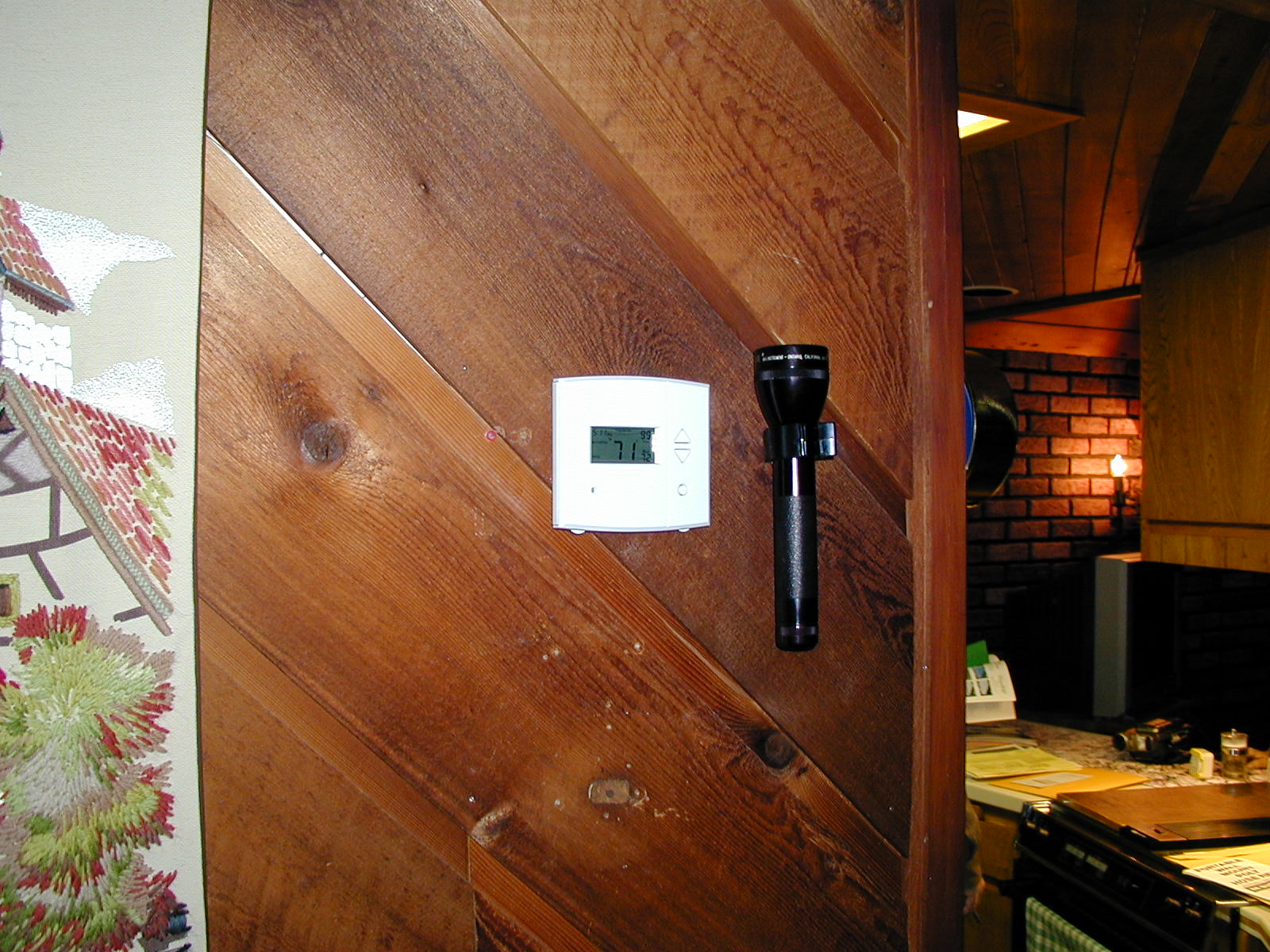The photograph captures the interior of a house, focusing on a section of a wood-paneled wall. The wood paneling, which dominates over half of the image, exhibits a rich texture with varying shades of brown. Mounted centrally on this paneling is a white square thermostat displaying a temperature of 71 degrees. Hanging on the same wood paneling is a black flashlight, positioned vertically with the bulb end at the top.

To the left of the wood paneling, the wall features a painted mural that depicts a colorful scene, including elements like a roof with shades of pink, red, green, and accents of white and gray, along with some bushes at the bottom. This painted area provides a stark contrast to the wood paneling.

On the right side, part of a brick wall is visible, complemented by what appears to be a light fixture, possibly another flashlight, positioned nearby. Additionally, there's a glimpse of a diagonal overhanging light. Below these elements, a wooden desk is cluttered with various objects including manila envelopes, yellow papers, assorted tools, and a glass of water, capturing the lived-in and functional essence of the room.